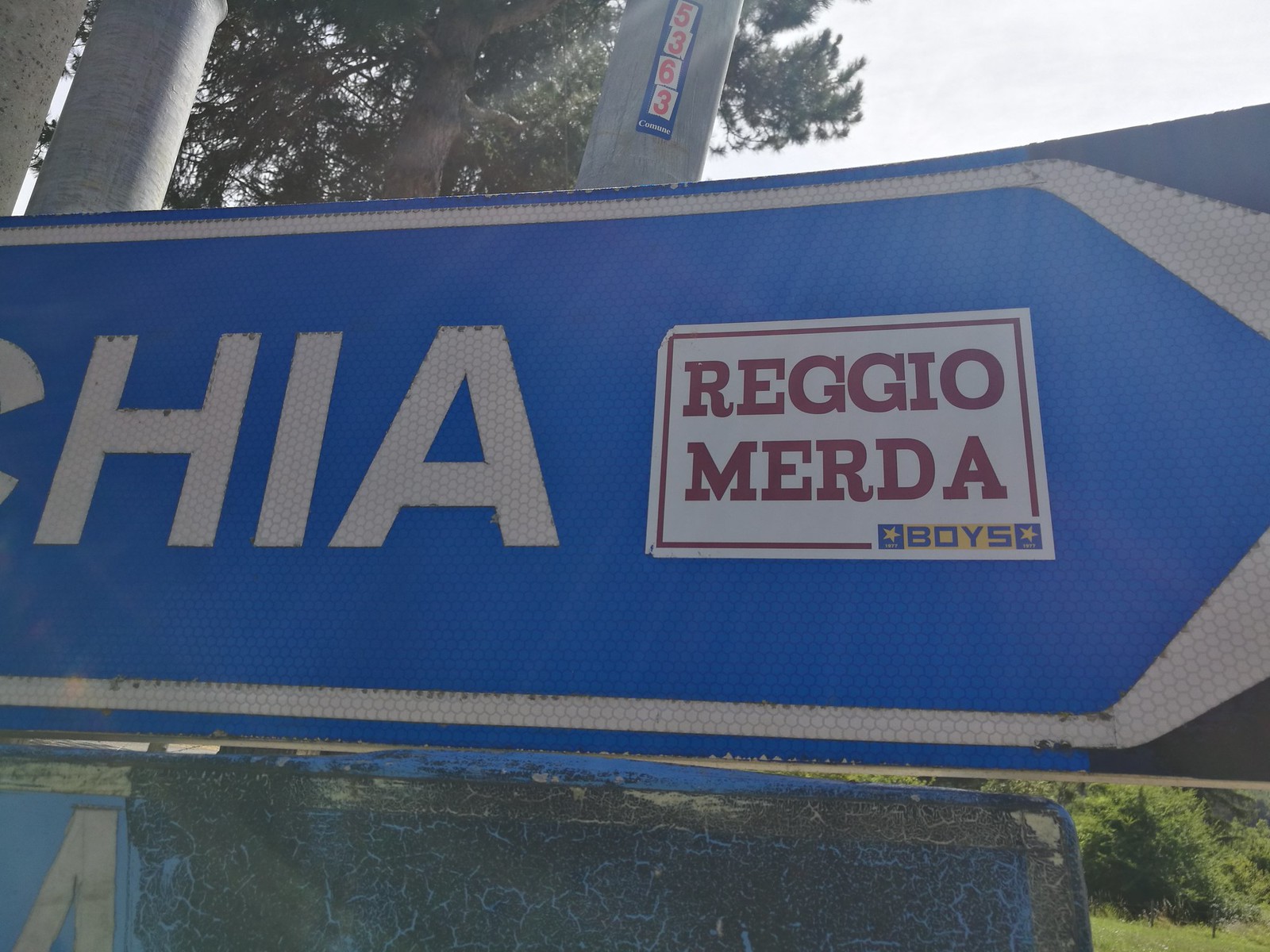The image features a blue street sign with the partially visible name "HIA" and a number "5363" taped onto the metal pole. Adorning the sign is a sticker with red text reading "Reggio Merda," followed by two yellow stars and the word "BOYS" beneath it, which might be an advertisement for a local election. Behind the sign, there are green bushes and trees, indicating that the image was taken in a real-life outdoor setting.